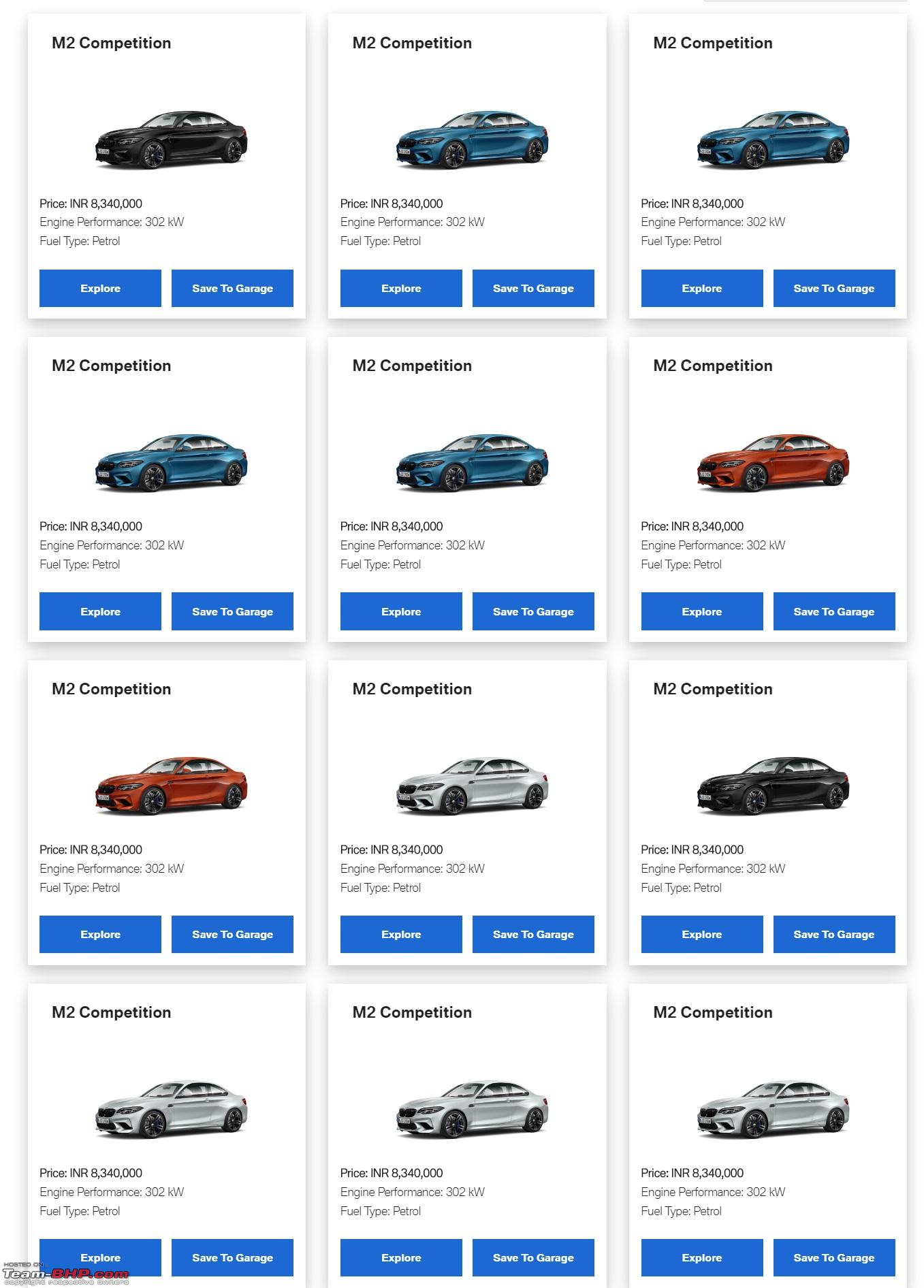**Detailed Caption:**

The image showcases a grid layout featuring twelve luxury sedans, arranged systematically in three columns and four rows. Each car is presented within its own box, with a bold black headline at the top of each box reading "M2 Competition." Despite slight variations in color, all cars appear to be of the same model. 

In the first column, the cars are predominantly black, while the second column features blue cars. The third column presents cars in a shade of blue that may be slightly different from those in the middle column. The first row displays a black, a blue, and another blue car from left to right. Moving down, the second row includes a blue, another blue, and a red car. The third row features a red, a silver, and a black car. Finally, the fourth row showcases three silver cars.

Each car's box contains detailed information beneath the image, listing the price as $8,340,000 (currency unspecified), engine performance at 302 kW, and petrol as the fuel type. Additionally, there are two blue buttons under each car: one labeled "Explore" and the other "Save to Garage."